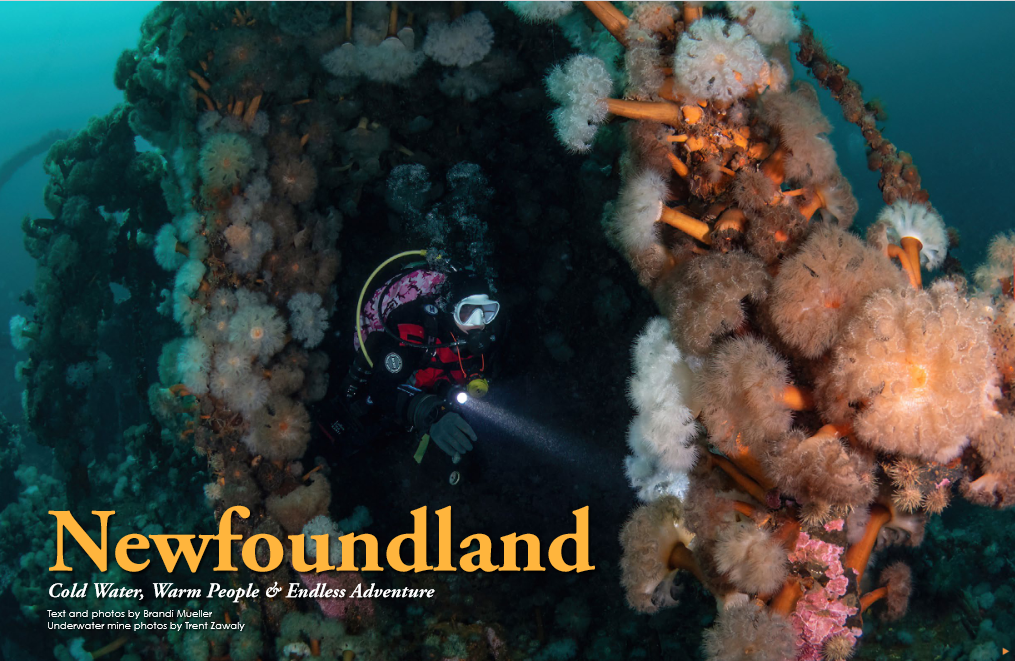The image is a horizontally aligned rectangular underwater photograph that resembles a poster or advertisement. In the lower left corner, bold yellowish-orange letters spell out "Newfoundland." Below that, smaller white text reads, "Cold water, warm people, and endless adventure." Tiny white text beneath it credits Brandi Mueller for the text and photos, and Trent Zawily for the underwater mine photos. The main focus of the image is a scuba diver, situated slightly left of center, who is using a flashlight to illuminate the vibrant underwater scene. The diver, dressed in red and black gear with a noticeable yellow hose, has their light trained on one of many fuzzy white and brown coral formations that appear almost pink. These colorful coral clusters form an archway structure that surrounds the diver, extending above and beside them. The background features more rocks, plants, and additional coral formations, creating a vivid and immersive underwater environment.